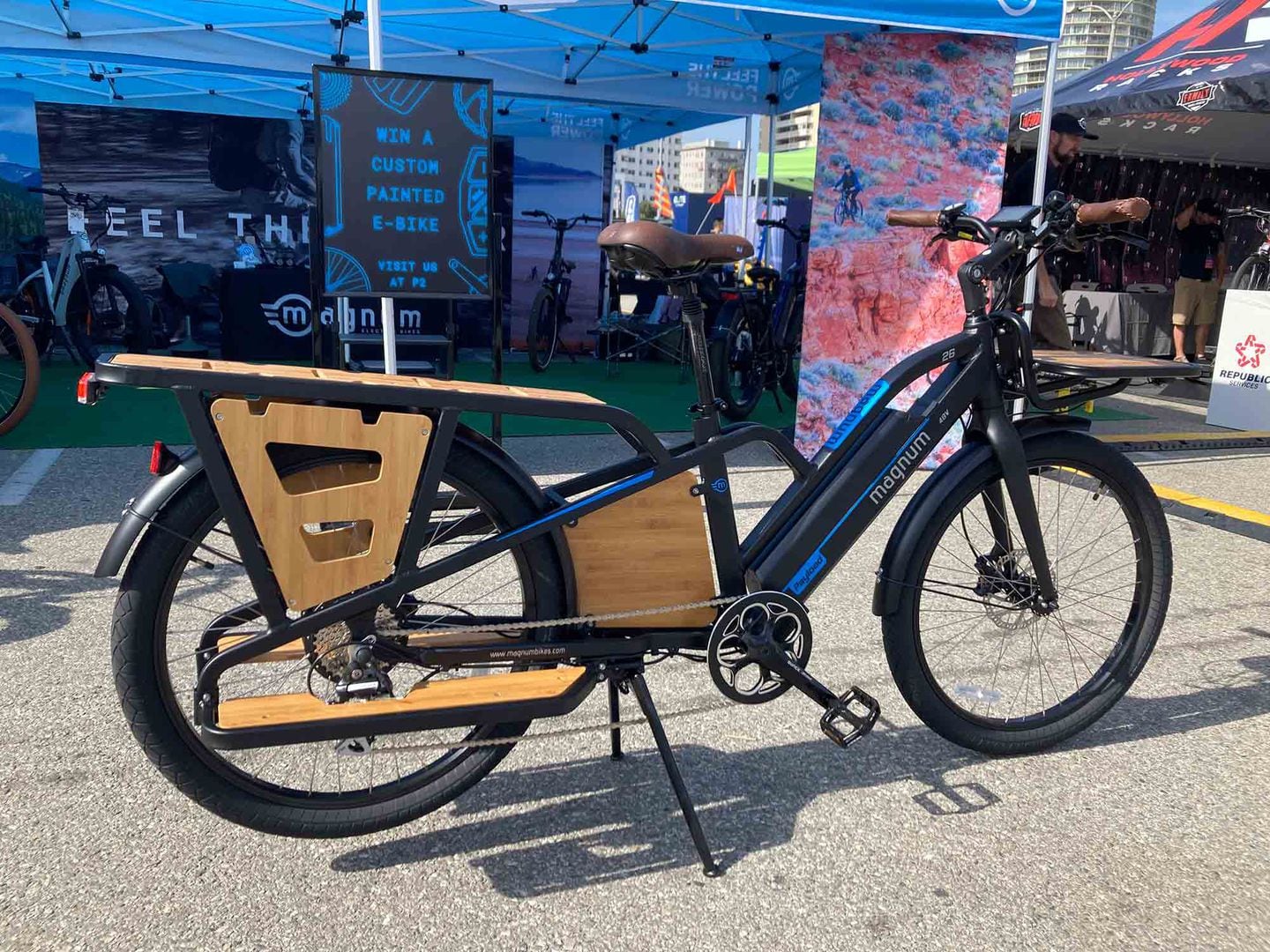The detailed image shows a custom-painted black electric bicycle with blue accents parked in front of a tent on a boardwalk by the beach. The bike features unique design elements, with racks at the back made from black plastic or metal with wood inserts, as well as wooden running boards behind the pedals for passenger footrests. The bike's frame includes wooden panels that evoke the structure of a motorbike. The back end of the bike is elevated on two stands, while the front wheel rests on the gray asphalt surface, casting a clear shadow under the bright sunlight. Behind the bike, a blue sign reads, "Win a custom-painted e-bike," with an accompanying image and the tagline "Feel this." In the background, there are several bicycles and pop-up tents, presumably for bike rentals or a display, adding to the lively beach setting.